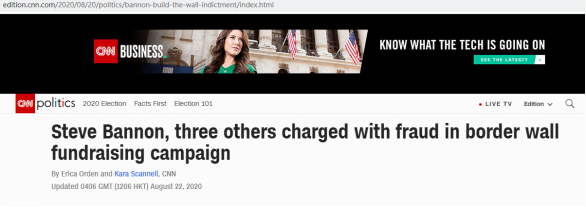The image is a screenshot capturing the upper portion of a CNN website, likely from a desktop or laptop display. At the top, a black banner spans across the screen. In the center of the banner, there is a photograph of a young woman with brown hair, dressed in a green shirt, standing in front of a federal building characterized by its stone facade, pillars, and American flags.

To the left of this image, the text "CNN Business" is displayed alongside the CNN logo, which is a red square bearing the white "CNN" lettering. Below this, the tagline reads, "Know what the tech is going on." Another banner beneath them states "CNN Politics, 2020 Election, Facts First."

Dominating the lower section of the screenshot is the headline of the main article, written in large black text against a white background: "Steve Bannon, three others charged with fraud in border wall fundraising campaign."